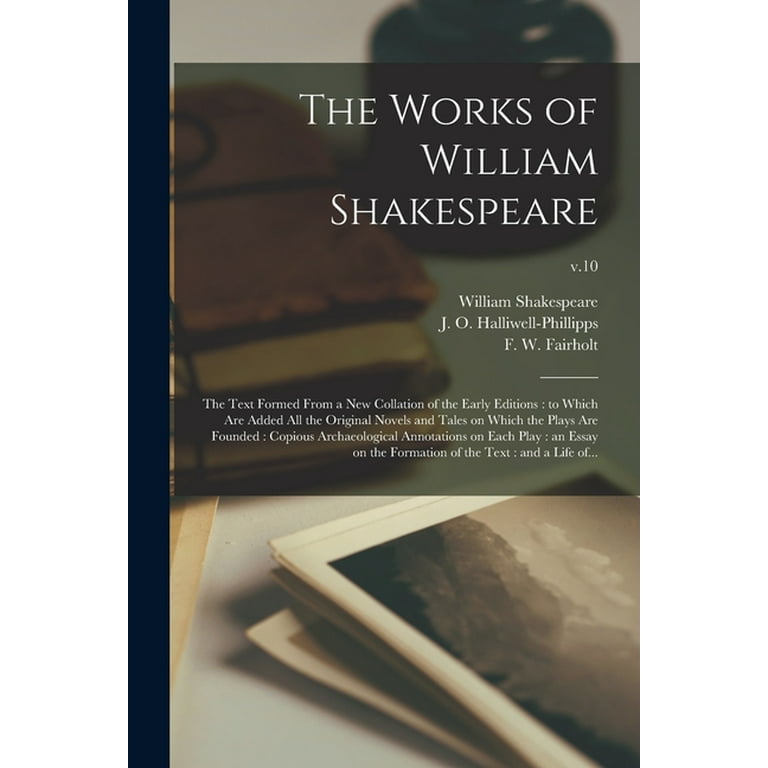The front cover of this book features a slightly blurred background that resembles the top of a desk, adorned with various items that evoke a sense of antiquity. Scattered across the desk are several old photographs, with one depicting a scenic view of clouds and mountains, as well as an old book or notebook and a cylindrical object that might be an inkwell, positioned at the top right. On the lower right corner, there are stacked photographs bordered in white.

Dominating the left-hand side of the cover is a black or bluish stripe, likely representing the book's binding. Centrally placed is a semi-transparent black textbox, through which elements of the desk are faintly visible. Inside this textbox, the title "The Works of William Shakespeare" is prominently displayed in bold white lettering, with "Volume 10" denoted beneath it. The authors William Shakespeare, J.L. Haywood Phillips, and F.W. Fairholt are listed in smaller white text below the title. Additional text describes the contents as a new collection of early editions, including original novels and tales on which Shakespeare's plays are based, as well as extensive archaeological annotations and essays on the formation of the text and Shakespeare's life, though the details trail off with ellipses. This intricate design sets the stage for a scholarly work on Shakespeare's timeless creations.